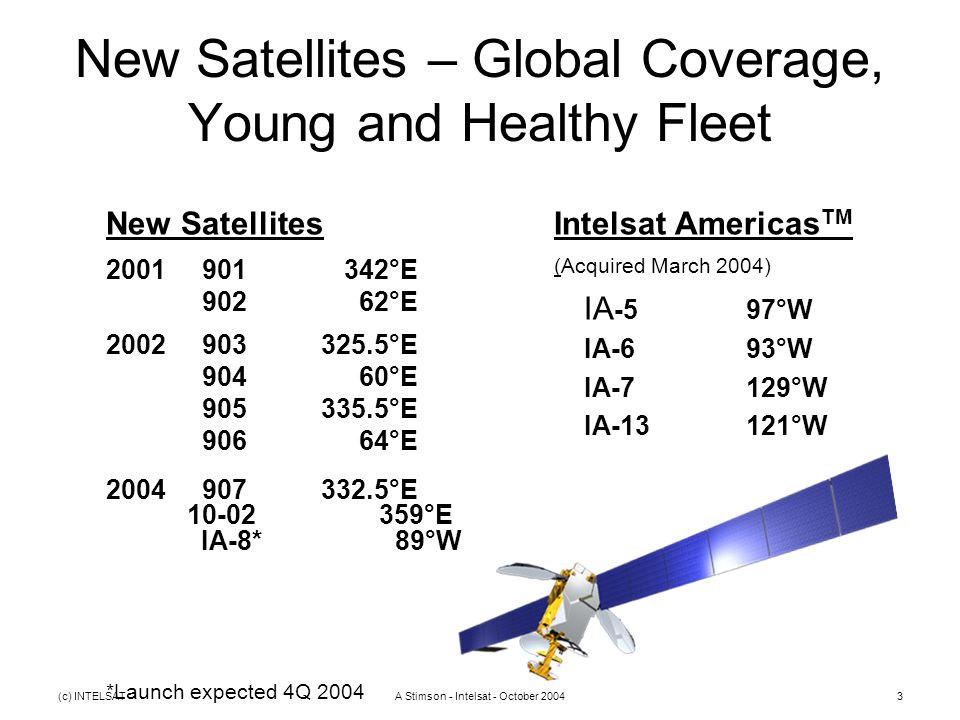This is a detailed infographic image providing information about new and existing satellites, their launch years, and their positions. The infographic prominently features the title "New Satellites, Global Coverage, Young and Healthy Fleet." The layout is organized into two main columns beneath the title. 

The left column, labeled "New Satellites," lists satellites launched in 2001, 2002, and 2004, including their geographical positions:
- For 2001: Satellite 901 is at 342 degrees east and Satellite 902 at 62 degrees east.
- For 2002: Satellite 903 at 325.5 degrees east, Satellite 904 at 60 degrees east, Satellite 905 at 335.5 degrees east, and Satellite 906 at 64 degrees east.
- For 2004: Satellite 907 at 332.3 degrees east and Satellite 1002 at 59 degrees east, with IA-8 marked with an asterisk at 89 degrees east.

The right column details the Intelsat Americas acquisitions, noting they were acquired in March 2004. It lists satellites AI5, AI6, AI7, and AI13 with their respective positions:
- AI5 at 97 degrees west
- AI6 at 93 degrees west
- AI7 at 129 degrees west
- AI13 at 121 degrees west

Beneath these columns, there is a computer-generated image of a satellite. The satellite features a white and gold central body, with two long blue reflective solar panels extending from its sides.

At the bottom of the image, it's noted that an Intelsat launch is expected in the fourth quarter of 2004, sponsored by Stimson Intelsat as of October 2004.